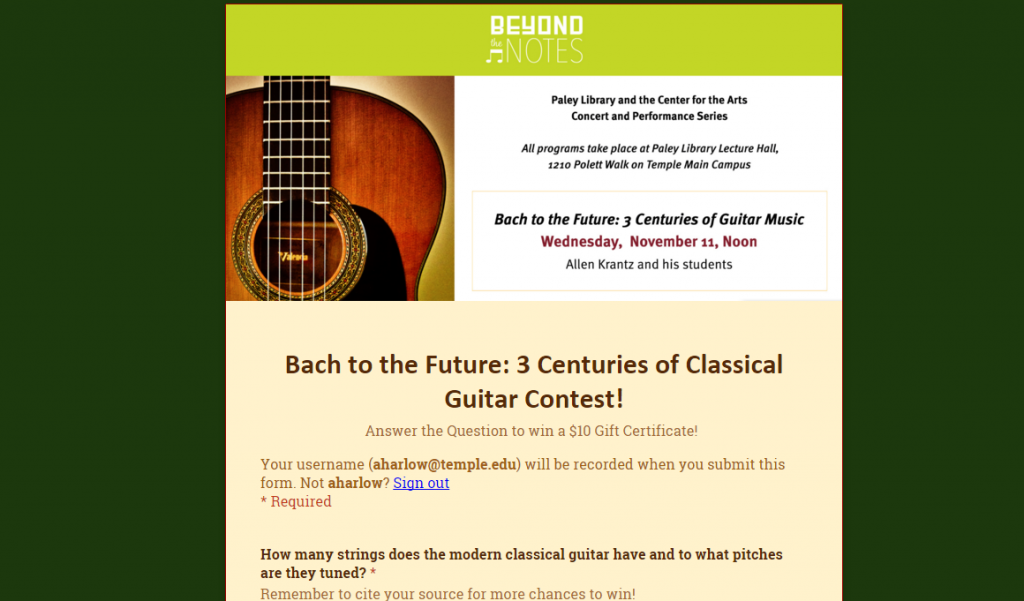The caption for your image can be cleaned up and detailed as follows:

---

The website appears to be called "Beyond the Notes." It features a dark hunter green color scheme on both sides, with a lighter green section in the middle at the top. The words "Beyond the Notes" are prominently displayed in this lighter green area. 

Beneath this title, positioned on the left side, there is an image of an acoustic guitar. On the right side of the image, the text reads: "Paley Library and Center for the Arts Concert Performance Series." Additional information is provided, stating, "All programs take place at Paley Library Center Lecture Hall, 1210 Holett Walk, Temple Main Campus."

The event advertised is titled "Walk to the Future: Three Centuries of Guitar Music," scheduled for Wednesday, November 11th at noon. Featured performers include Allen Krantz and his students, with a program named "Bach to the Future: Three Centuries of Classical Guitar."

The announcement also invites participants to answer questions for a chance to win a $10 gift certificate. One of the questions asks, "How many strings does a modern classical guitar have and to which pitch are they tuned?"

Users are instructed to submit their answers while logged in, as noted by the username example "aharlow@temple.edu." The form submission will be recorded, and the "Sign Out" link is highlighted in blue and underlined. Additionally, there is a required field marked with an asterisk.